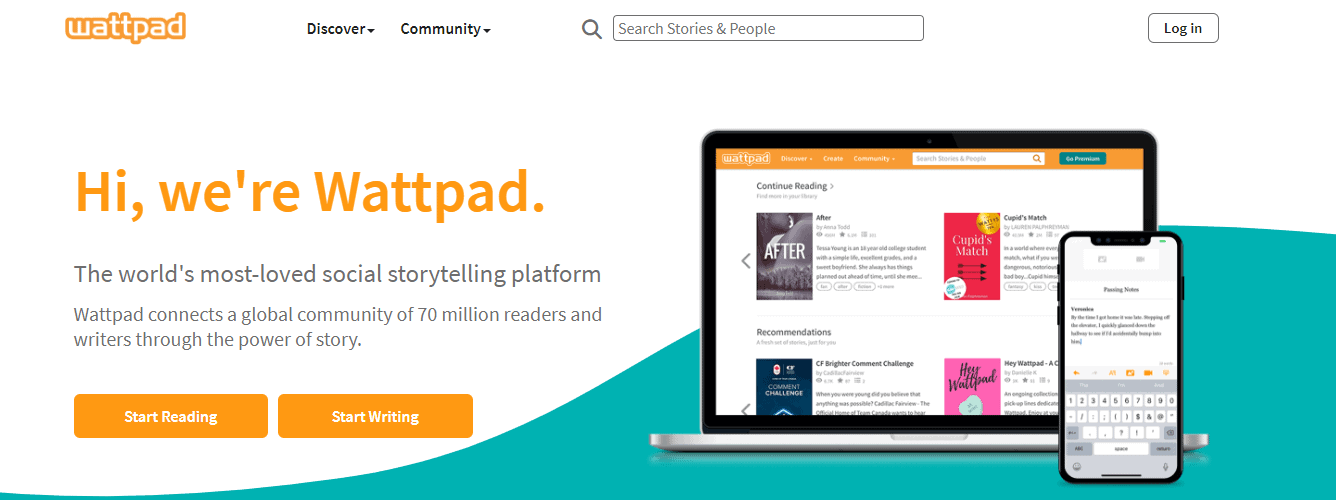The image is a screenshot of the Wattpad website. At the top left, the Wattpad logo is prominently displayed in orange with white text outlining "W-A-T-T-P-A-D." To the right of the logo, there is a navigation menu with "Discover" and "Community" options followed by a centrally-located search bar. The search bar, framed by a magnifying glass icon, includes the placeholder text "Search stories and people." On the far right of the navigation bar, a rectangular white button labeled "Login" is situated.

Below the navigation bar, a welcoming message reads, "Hi, we're Wattpad," followed by a subtitle, "The world's most loved social storytelling platform." The text highlights Wattpad's role in connecting a global community of 70 million readers and writers "through the Power of Story."

Beneath the introductory message, two prominent orange buttons invite users to either "Start Reading" or "Start Writing." Adjacent to these buttons is an image of a laptop displaying four story covers, resembling book covers, emphasizing the visual nature of the platform. Overlaying the laptop image is a cell phone displaying a keyboard and some text, signifying that Wattpad is also accessible via mobile devices.